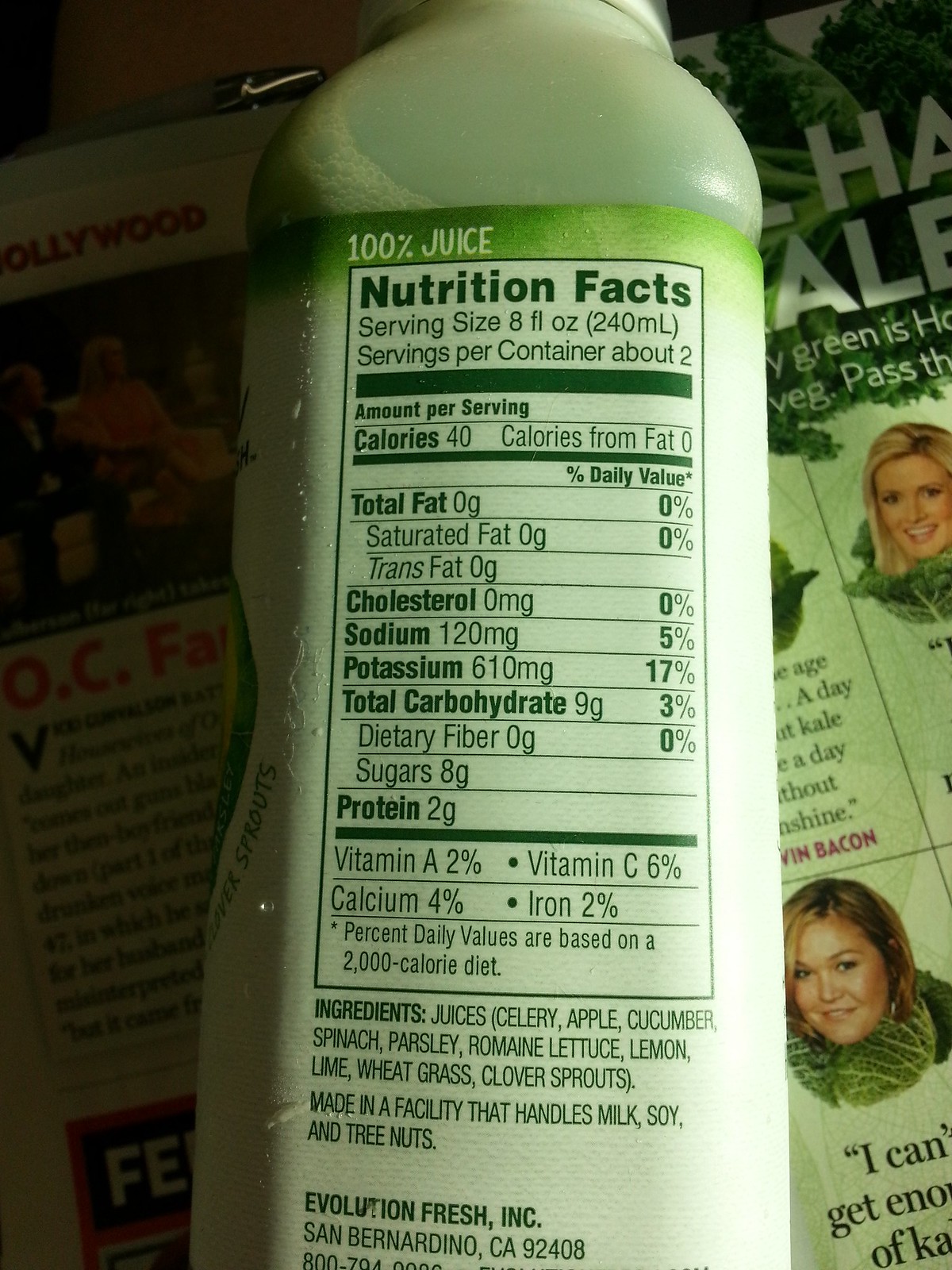This detailed photograph showcases a close-up view of the side of a transparent green juice bottle, prominently displaying its nutritional label. The top of the label states "100% juice," followed by detailed nutritional facts: 40 calories, 0g total fat, 120mg sodium, 610mg potassium, 9g total carbohydrates, 8g sugars, and 2g protein. The label also lists ingredients such as celery, apple, cucumber, spinach, parsley, romaine lettuce, lemon, lime, wheatgrass, and clover sprouts, and mentions that it is made in a facility that handles milk, soy, and tree nuts by Evolution Fresh Incorporated.

The juice is visibly green through the bottle, indicating its healthy, vegetal content. Alongside the bottle, the photograph captures part of a magazine. This contains images and quotes from various actresses, including Holly Madison, superimposed on pieces of cabbage, with the word "Hollywood" noticeable at the top. The visual composition suggests a context promoting healthy eating habits and juice consumption.